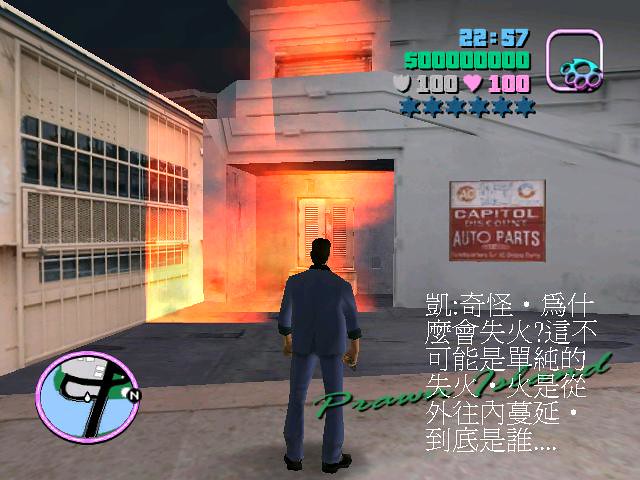The image depicts a screenshot from a video game resembling the Grand Theft Auto series, evidenced by the user interface elements such as a mini-map on the bottom left and detailed information on the top right, including time, money, health, armor, and wanted level. In the third-person perspective, the player-controlled character—a man—is standing outside a burning building at night. The building, clearly labeled as an auto parts store with signage on its exterior, is engulfed in flames primarily at the entrance and on the second floor. No other characters are visible in the scene. To the left of the auto parts store is a warehouse with visible windows, suggesting that both buildings are part of the same industrial complex.